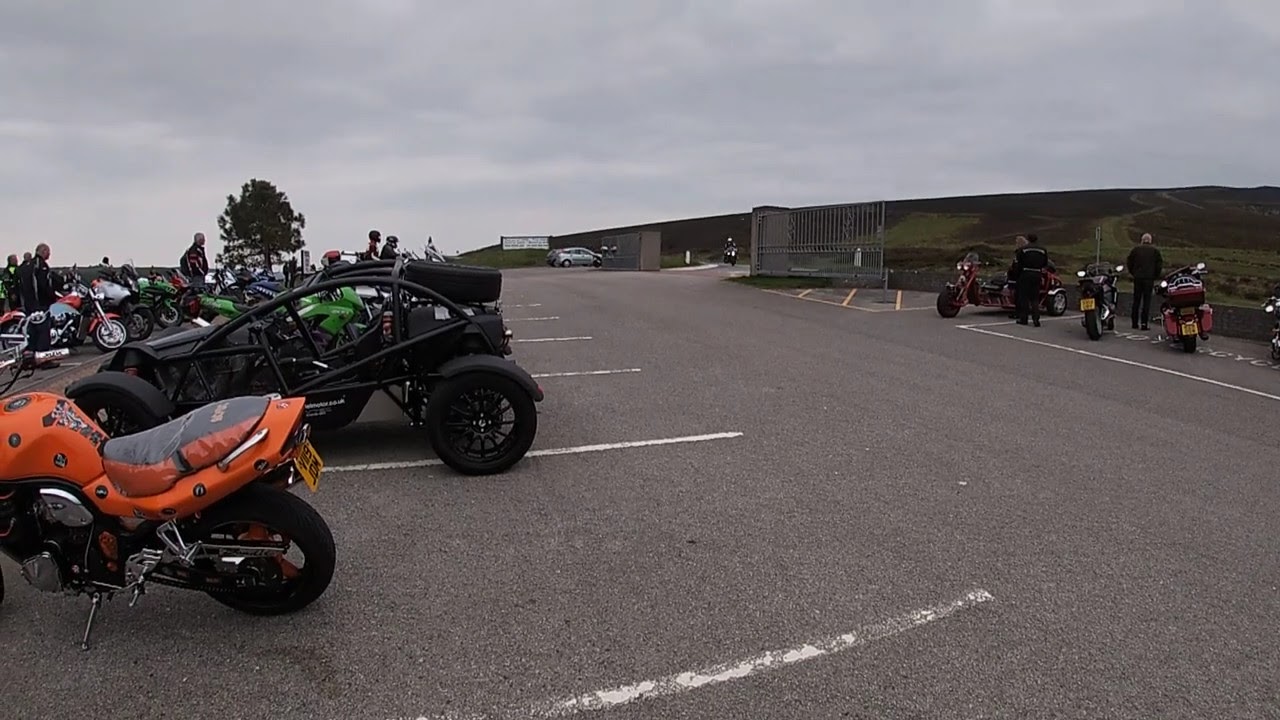In this detailed scene, the focal point is a large parking lot bustling with activity. Multiple motorcycles are lined up predominantly on the right-hand side; two men are seen standing next to their bikes, with their backs facing the camera. An open gate in the background reveals a motorcyclist riding through. On the left, an eye-catching bright orange motorcycle is situated beside an advanced dune buggy. Several other vehicles, including sport utility vehicles and a gray station wagon, are visible around the lot. White lane markings are clearly seen on the paved surface. The horizon is dominated by large hills under an overcast sky, filled with gray clouds, indicating a potentially serene setting that resembles a park or perhaps a beach. A hint of a trail leading up one of the hills adds to this ambiance. The overall composition conveys a blend of a gathering spot for motorcycle enthusiasts amidst a picturesque landscape.